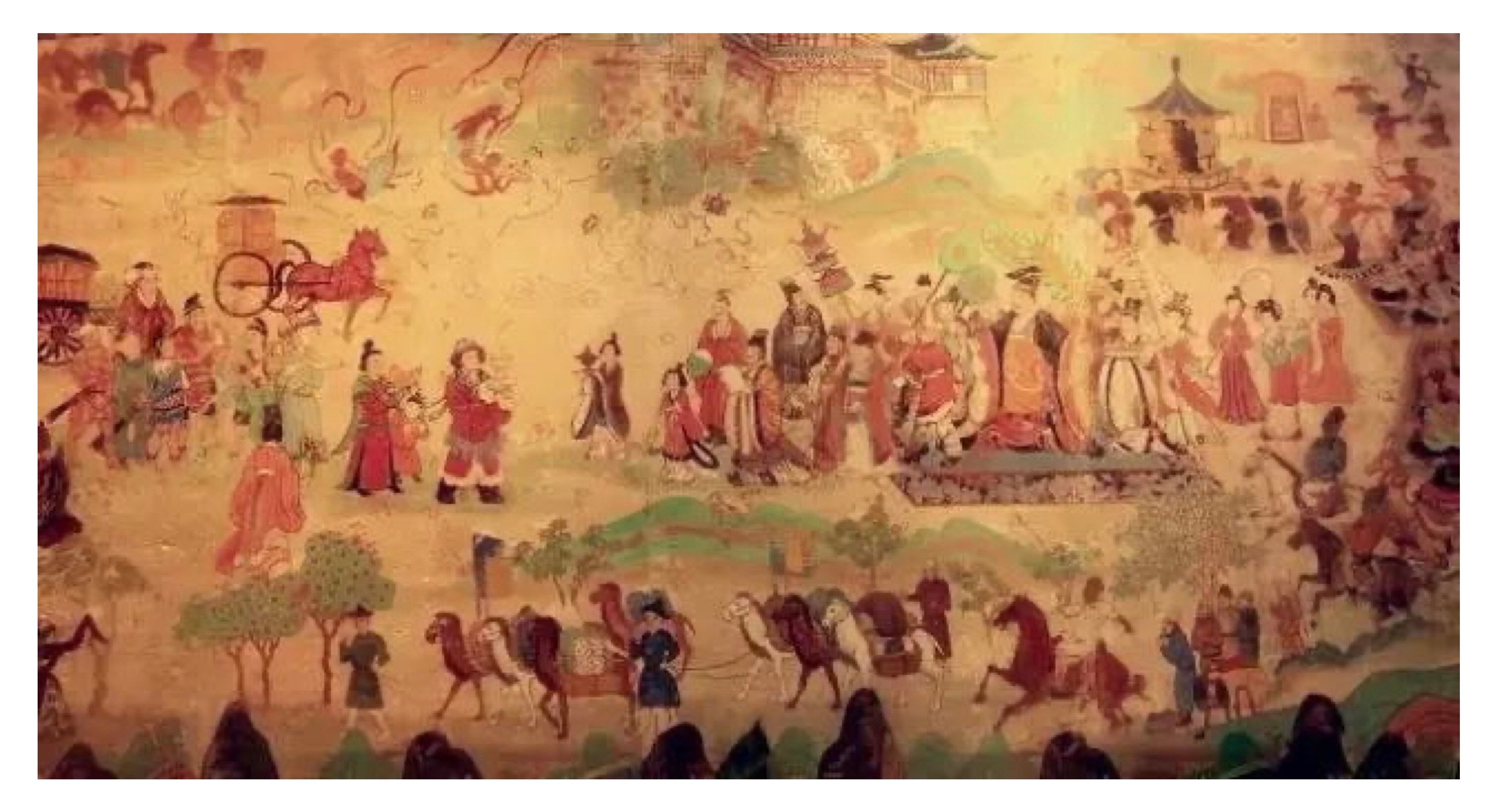This rectangular, horizontal painting appears to be an old Chinese artwork with a predominantly gold and yellowish-brown background, giving it an oxidized and faded look. At its heart, the painting features a central figure, likely a king or emperor, standing on a platform and adorned in a golden robe with brown accents around the shoulders. He is surrounded by his court, and clusters of people are gathered around him, fully engrossed in various activities.

To the left, a procession heads towards the emperor, including someone carrying a trophy and another individual playing an instrument. The bottom part of the painting depicts horses and camels, some adorned and carrying items on their backs, marching through the fields. Additionally, horse-drawn carriages can be seen making their way toward the center.

The scene is bustling with activity: groups of people in elaborate robes, trees scattered throughout, and various small houses and structures dotting the landscape. The artwork is rich in detail and color, with vibrant reds in the clothing and shiny browns in the horses, amidst the overall beige, gold, and yellowish hues. Overall, the painting presents an intricate and lively depiction of a historic moment filled with cultural significance.